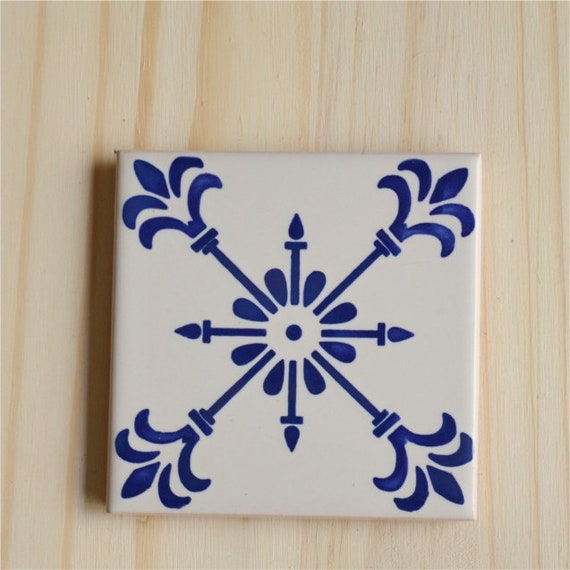This perfectly square image showcases a single, white decorative tile with an intricate blue fleur-de-lis design. The tile features a pattern which combines traditional floral and teardrop motifs in a symmetrical X shape. Extending from each of the four corners, blue lines connect to the center where a delicate, flowery pattern with a dot is situated. The background is a very light wood surface with subtle grain details, adding contrast to the off-white tile and emphasizing its delicate blue artwork. The tile is slightly off-center, positioned towards the bottom-right of the image, with a minor imperfection in the upper-left corner. This beautifully detailed image leaves a sense of ambiguity regarding the tile's purpose—whether it be for a floor, wall, or perhaps as a decorative coaster—highlighting its versatile appeal.